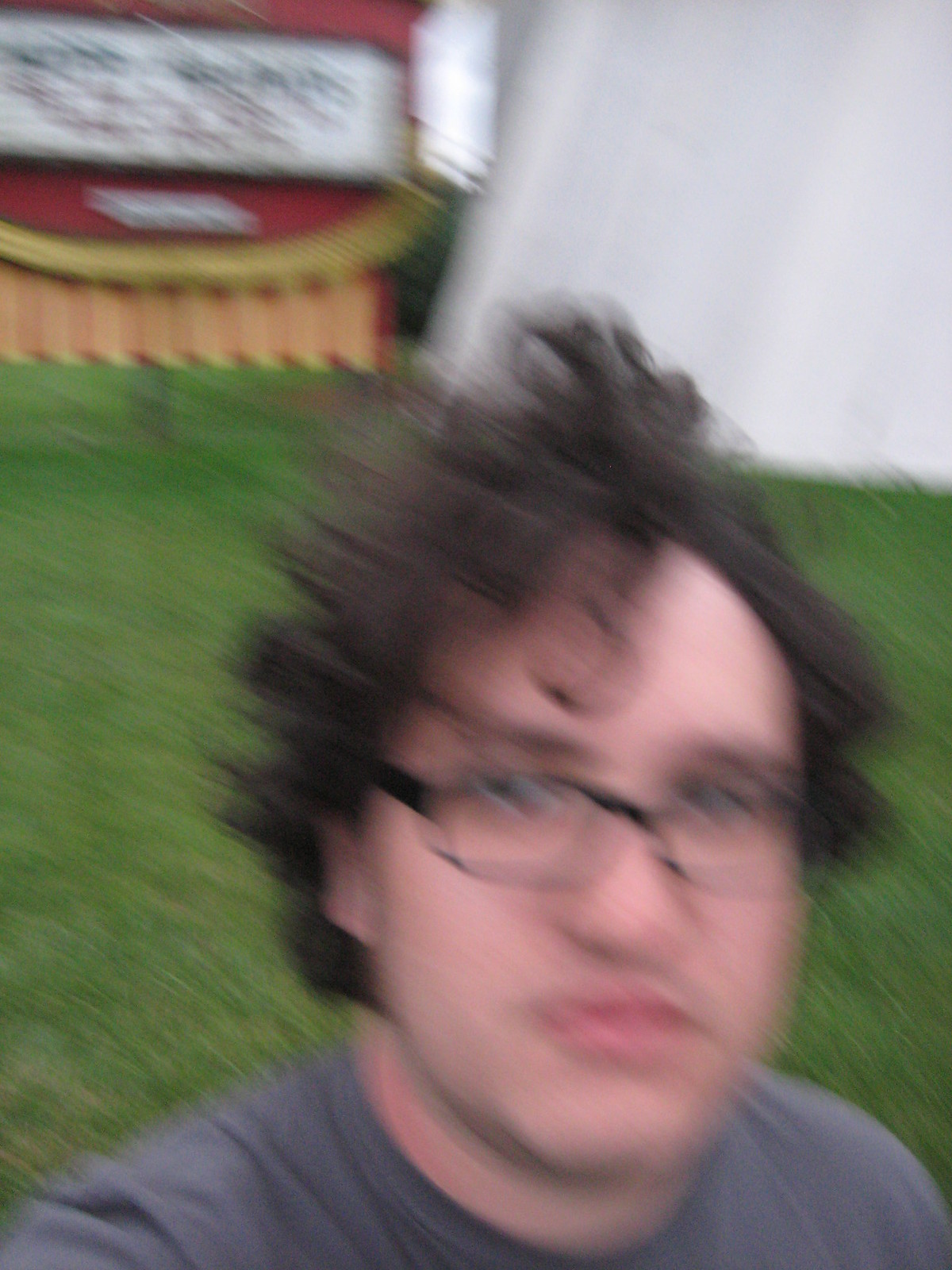A blurry color selfie shows a fair-skinned man with dark curly hair, bushy eyebrows, and full lips. He is wearing black-framed glasses and a gray round-neck t-shirt, and appears to have some stubble on his mustache area. The photo is taken outdoors, possibly at a fair or festival. Behind him, there is manicured green grass, a large white structure, and a colorful, intricate sign with peach, red, gold, and white elements, which appears to give information about an upcoming show or performance but is difficult to read due to the blur. The scene suggests a lively, public setting with large tents and possibly other buildings.